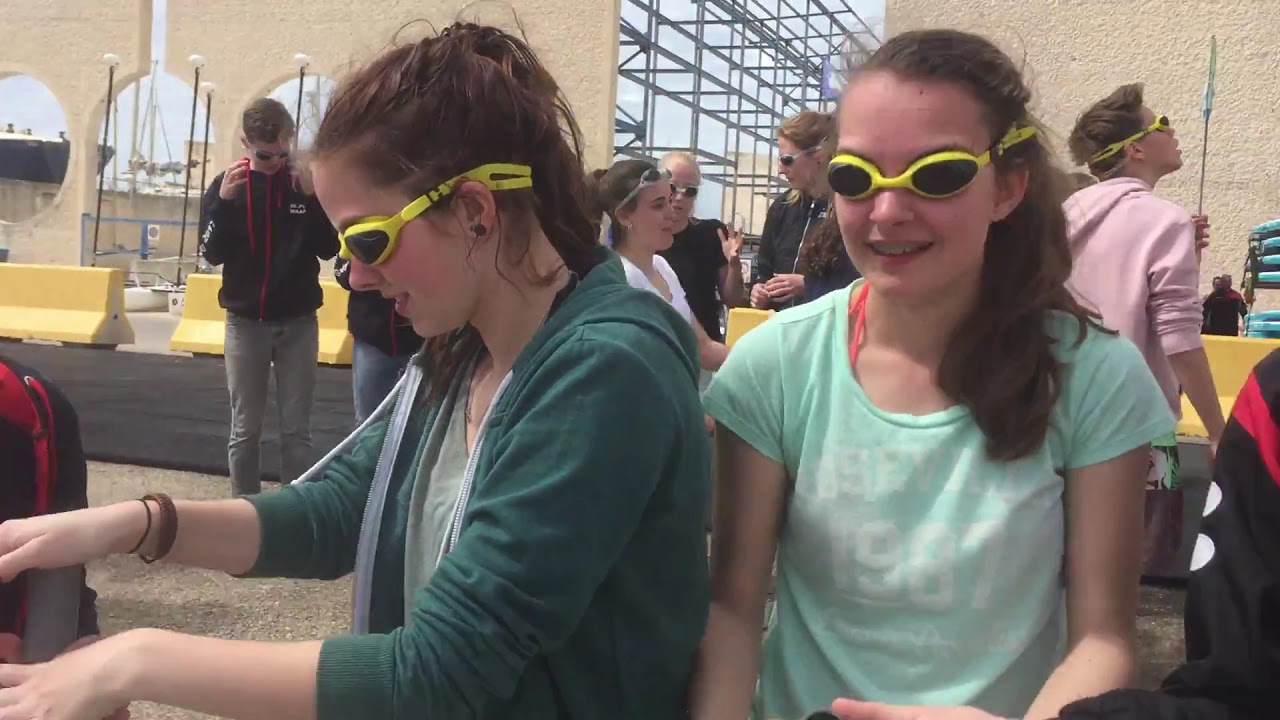The image depicts a group of children outdoors, engaged in what seems to be some sort of coordinated activity. At the forefront are two younger girls, both with brown hair tied back, wearing brightly colored yellow swim goggles with black lenses that give them an almost whimsical, alien-like appearance. One of the girls is smiling and dressed in a green short-sleeve shirt that reads "1987." Beside her, the other girl also smiles, donning a green hoodie over a light green shirt. The vivid and varied colors in their attire contrast with the background.

In the distance behind them, there are approximately five more children, also wearing goggles of either gray or yellow hues and dressed in an assortment of colorful shirts, including pink, white, black, dark green, and light green. Farther back stands a concrete yellow and black divider, shielding them from vehicular traffic and suggesting a construction zone, underscored by the visible scaffolding structures and tan walls behind it. The sky above appears overcast with patches of blue peeking through, contributing to the cool tone of the scene. This lively and intriguing snapshot captures a moment filled with youthful energy and the curiosity of outdoor exploration.